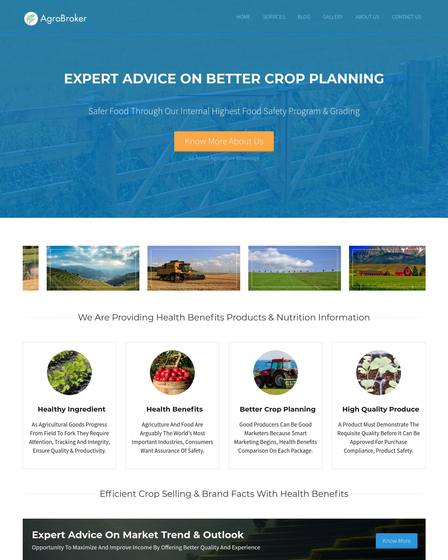The image features a striking and organized layout designed to convey agricultural expertise and food safety. Starting at the top, a serene blue background fades into view, punctuated by a fence running alongside a walking path. In the upper left corner, a small white circle appears, adjacent to which the phrase "Agro Broker" is written. Dominating the upper section, bold white capitalized text reads: "EXPERT ADVICE ON BETTER CROP PLANNING, SAFER FOOD THROUGH OUR INTERNAL HIGHEST FOOD SAFETY PROGRAM IN GRADY." 

Beneath this headline, an orange box contains a subtle invitation in light text: "Know more about us." Following this, the content is divided into distinct square sections. The first square presents a picturesque scene of majestic mountains under the sky, with lush green hills in the foreground. The following square depicts a tractor at work in a vast field, suggestive of efficient farming practices. Next, the image showcases a pristine expanse of bright green grass under a sky adorned with clouds, symbolizing fertile and healthy soil. The final square in this series features another red tractor set against a vibrant green field, emphasizing modern agricultural equipment.

Further down, accompanying labels elucidate the images, enhancing their meaning. The first, titled "Healthy Ingredient," displays an assortment of green vegetables. Next, a barrel filled with ripe tomatoes is captioned "Health Benefits." Below this, an image of a tractor in a field is paired with the label "Better Crop Planning." Finally, an image depicting delicate white flowers or produce is captioned "High Quality Produce."

At the very bottom, the detailed and informative caption concludes with a reassurance of ongoing professional support: "EXPERT ADVICE ON MARKET TREND AND OUTLOOK." This well-crafted image delivers a clear message about the dedication to quality, safety, and expertise in the agricultural sector.